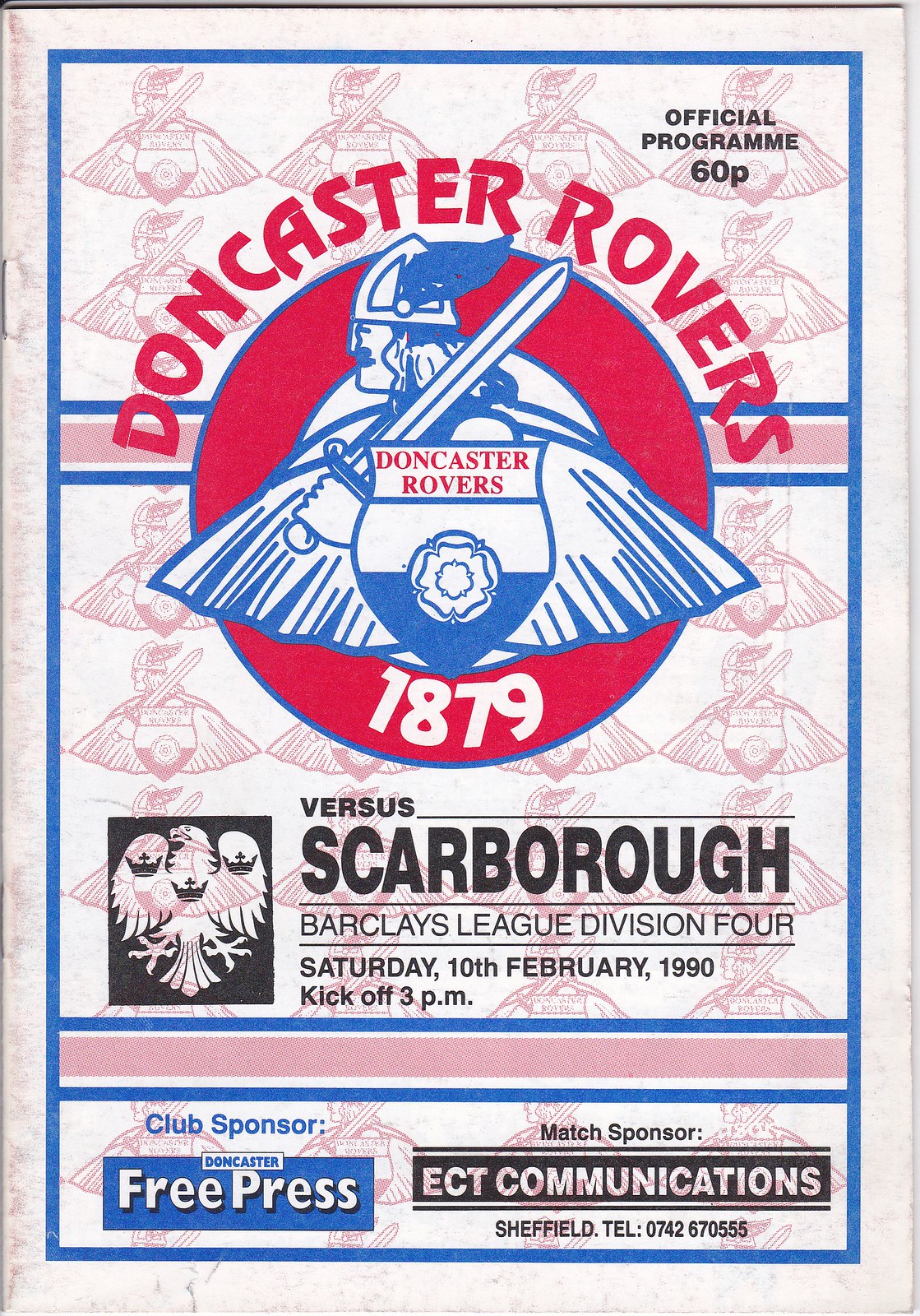This is a detailed description of the cover page of a Doncaster Rovers Official Program for a soccer match. The background features a Doncaster Rovers logo, a red-outlined knight or gladiator figure in a Viking-style helmet, holding a sword and cape. The background images are arranged in a grid of four horizontally and seven vertically. In the top right corner, "Official Program 60p" is printed in black text. Dominating the center is a large version of the logo inside a red circle, with the text "Doncaster Rovers 1879" above the circle in red font. The large logo differs from the background logos by having a blue outline.

Below this central logo, the information for the match is presented: "Versus Scarborough Barclays League Division 4, Saturday, 10th February 1990, kickoff at 3 p.m." To the left of this text is a crest with a falcon in a black box with white outlines, indicating Scarborough's emblem. 

Towards the bottom, the club sponsor and match sponsor information is displayed. On the left side, it says "Club Sponsor: Doncaster Free Press" in blue font within a blue box. On the right side, it reads "Match Sponsor: ECT Communications" in a black font followed by contact information: "Sheffield Tel: 0742 670555" in a black box with white text. A blue and red-bordered divider separates these segments.